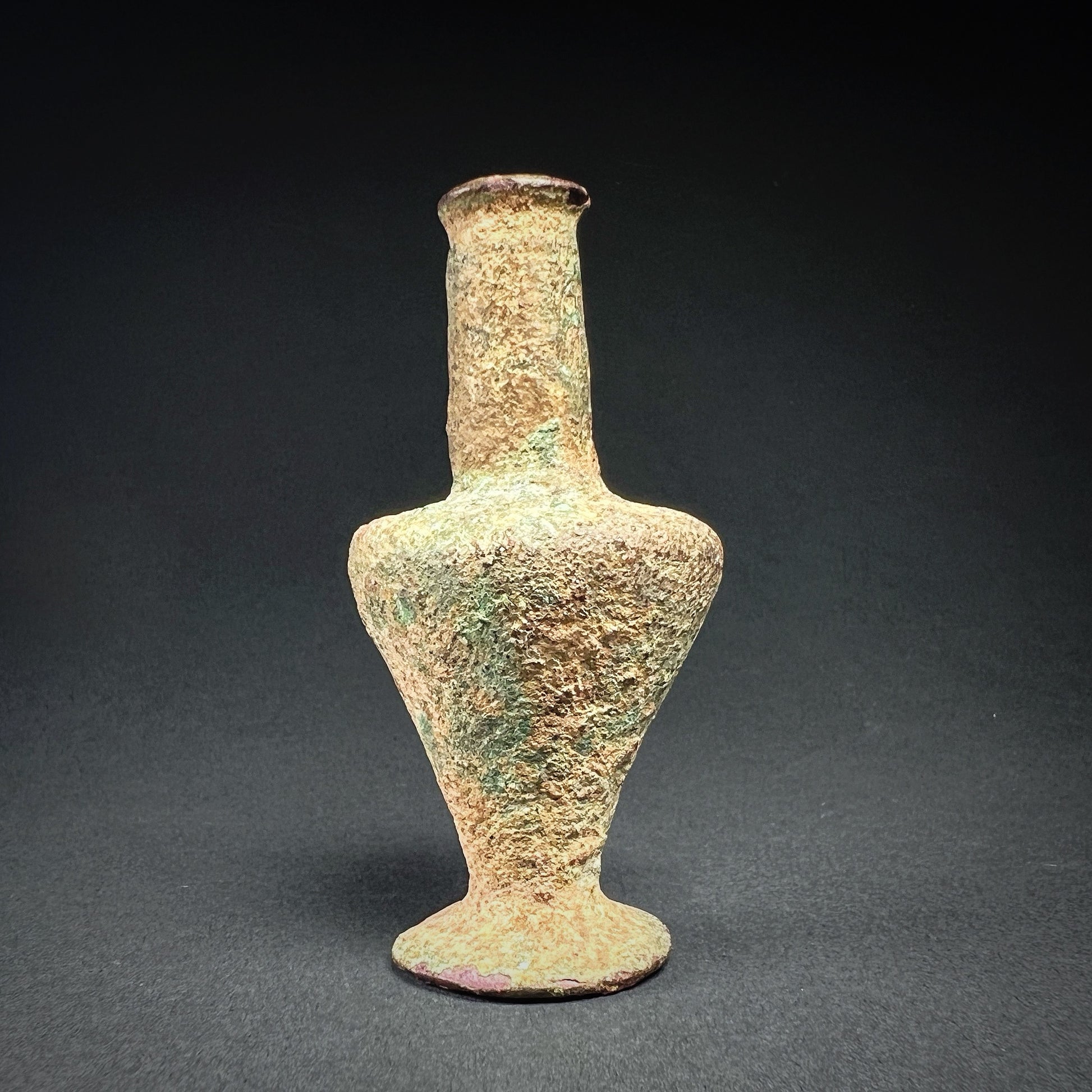This image features an ancient artifact, possibly a vase or container, with a distinctive and weathered appearance. The object has a rough texture, suggesting it may have rested in the sea for an extended period, leading to its encrusted surface, possibly with barnacles or other marine detritus. The vase narrows into a cylinder at the top, flares outward in the middle to form a wider, vase-like shape, and then expands again into a circular cylinder base, allowing it to stand upright. The original color appears to be a dark brown, especially noticeable at the top portion, and it is currently displayed as if it were a museum piece on a felt surface under a bright light. The backdrop transitions smoothly from black at the top to gray, providing a stark contrast that accentuates the artifact's intriguing and ancient features.